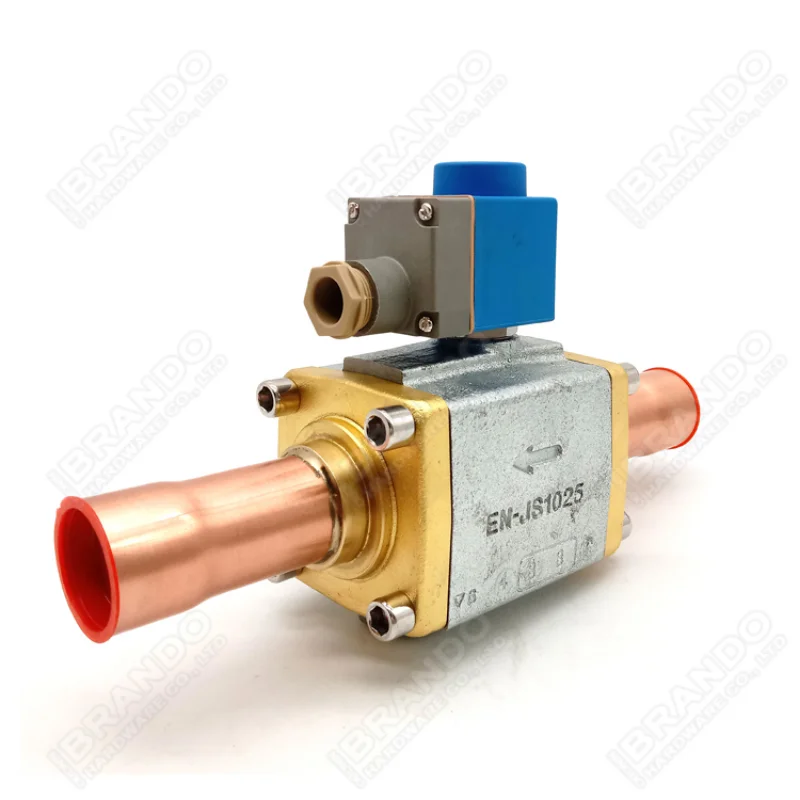The image depicts a device that appears to be a type of electronic or switch valve, likely used for plumbing or electrical conduit purposes. The central component is a cube-like metallic box, primarily silver in color, etched with the alphanumeric code ENJ81025 and featuring an arrow pointing left, indicating the direction of flow. The edges of this silver box are adorned with gold plates, and on either side, there are copper projections with red interiors.

Above the main silver box, there is a smaller blue and gray box, fitted with a hexagonal brown plastic nut that is likely a part of the valve mechanism. This smaller box has a single tube protruding from the top, possibly indicating a pneumatic switch function responsible for regulating pressure to open or close the valve below.

The background of the image contains diagonal watermarks featuring the text "Brando Brando Hardware Company Ltd," suggesting the manufacturer's branding. Additional features include screws that secure different parts of the device and gold trim on either side of the main base, contributing to its structural integrity and aesthetic detail.